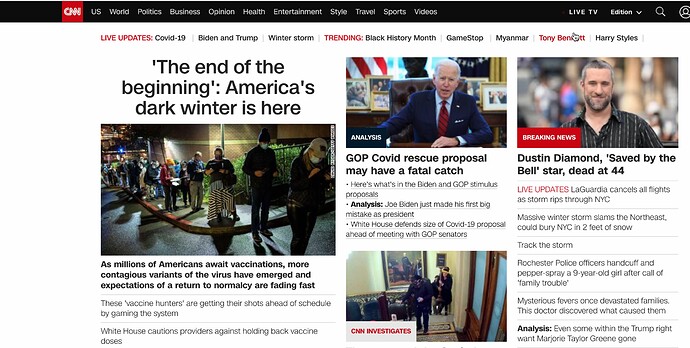**Detailed Caption:**

This image is a screenshot of the CNN website from a few years ago. It features a white overall background with a prominent black top navigation bar. The top bar includes the red CNN logo with white lettering, followed by menu options listed as: U.S., World, Politics, Business, Opinion, Health, Entertainment, Style, Travel, Sports, Videos, Live TV, a drop-down menu for editions, a search bar, and a profile icon for user sign-in.

Below the main navigation, there is a submenu with categories such as Live Updates, COVID-19, Biden and Trump, Winter Storm, Trending, Black History Month, GameStop, Myanmar, Tony Bennett, and Harry Styles. Notably, "Live Updates," "Trending," and "Tony Bennett" are highlighted in red font, while the rest are in black.

Highlighted news articles on the page include:
- "The End of the Beginning: America’s Dark Winter is Here," which discusses vaccines.
- "GOP COVID Rescue Proposal May Have a Fatal Catch."
- "CNN Investigates."

Additional stories on the page report:
- LaGuardia canceling flights due to winter storms slamming the Northeast.
- Rochester police officers handcuffing and pepper-spraying a nine-year-old girl.
- Analysis on intra-party desire for Marjorie Taylor Greene's removal from the Trump-right faction.

The screenshot also contains indicators that this page is not current: one of the breaking news stories announces the death of "Saved by the Bell" star Dustin Diamond at age 44, who passed away a few years ago, and the presence of live COVID-19 updates, which have since ceased. The mention of Black History Month trending suggests this was during February.